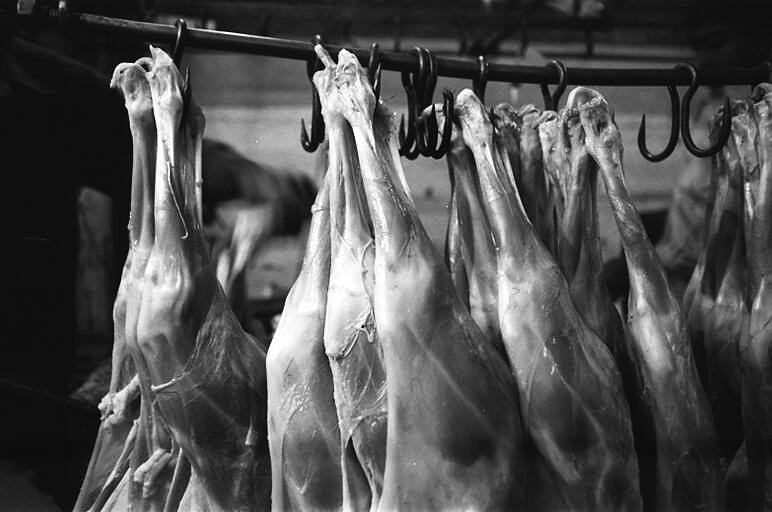In this detailed black and white photograph, several pieces of meat are hanging, likely from a meat processing plant or butcher's freezer. The meat, appearing to be the lower leg or thighs of skinned birds such as chickens or possibly turkeys, is suspended upside down from dark-colored hooks attached to a metal rod that runs across the top of the frame. The focal point of the image clearly shows four pieces in the foreground, with additional obscured pieces visible behind them, and another visible to the far right. The background is blurred, revealing indistinct shades of dark and light gray with shadowy objects, enhancing the prominence of the hanging meat. The photo evokes the industrial setting of meat processing, with the carcasses likely prepared for distribution.